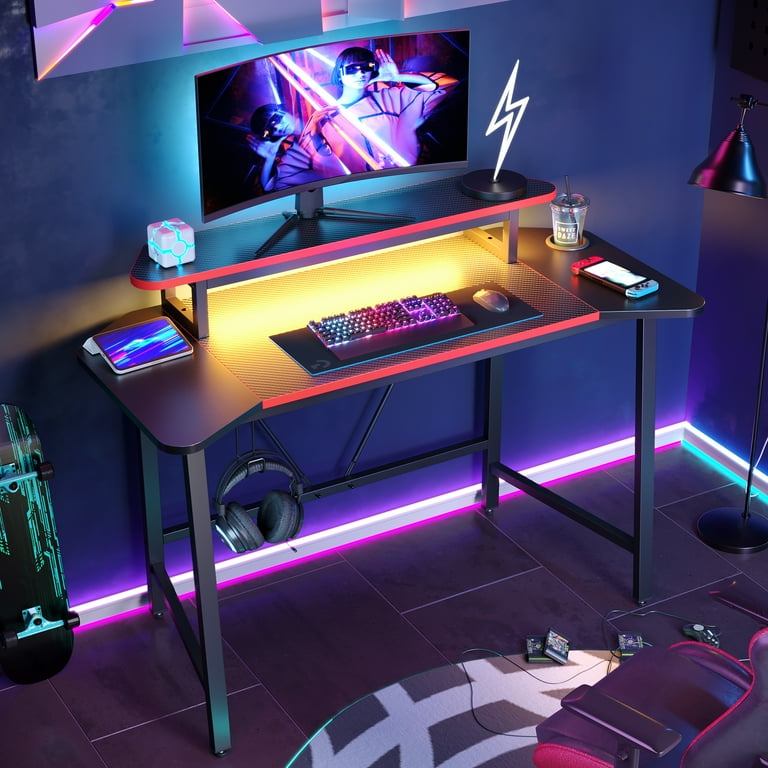This photograph captures an engaging and atmospheric PC gamer's setup in a dimly-lit room accented by various neon lights. Centered on a black, metal-framed, two-tiered desk, the primary feature is a slightly curved widescreen monitor displaying two men in a neon room. Flanking the monitor on the first tier are a small, decorative portal-like box on the left and a lightning bolt memorabilia piece on the right. The lower tier of the desk hosts a fluorescent light-up keyboard, mouse, and wrist protector, with a cup holder containing a drink cup and a Nintendo Switch to the right. A tablet and a light-up cube with glowing lines sit on the left side of this tier.

An impressively rounded desktop PC sits nearby, reflected in the room’s softly radiant backlighting which transitions from white at the top to pink at the bottom, and blue on the opposing wall. The desk itself is augmented by various fluorescent lights lining its edges and features a colorful rug beneath it with black and white circular patterns. A pair of large headphones hangs beneath the desk, and a black-and-green skateboard leans casually against the left wall. Strewn about the room's floor are retro Sega Genesis cartridges and a bootleg controller, adding a nostalgic touch.

The setup includes a dark gray and pink chair centrally positioned in front of the desk. To the right-hand corner of the room, a lamp casts additional ambient light, enhancing the overall luminous aesthetic of this immersive gaming environment.